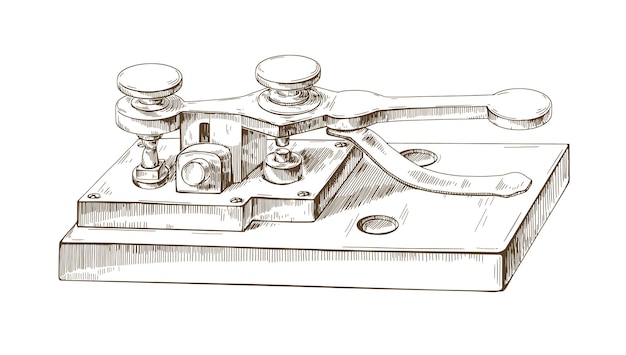This black and white, textured illustration appears to be a detailed sketched drawing of a Morse code telegraph device. The contraption is mounted on a flat, rectangular base that resembles wood, characterized by its multiple shaded areas to create a sense of depth and texture. Notably, there are two circular holes positioned towards the right center of this base, enhancing its intricate design. 

On the left section of the base, another smaller, rectangular layer is screwed down, using at least five or six visible screws at the corners, indicating solid construction. This smaller, raised platform supports a metal lever mechanism extending to the right. The lever, detailed with texture to suggest a metallic composition, functions by pressing down to produce the characteristic clicking sound associated with Morse code transmission.

Additionally, there's a pole-like piece situated centrally with a small, curved piece attached at the end, resembling the operation mechanism of the telegraph. This curved piece likely functions as the tapping component, striking against the underlying surface to generate the distinct telegraphic clicks. Overall, the drawing shows a strongly detailed, vintage telegraph device designed for Morse code communication, with an emphasis on its sturdy, textured base and precisely illustrated mechanical components.